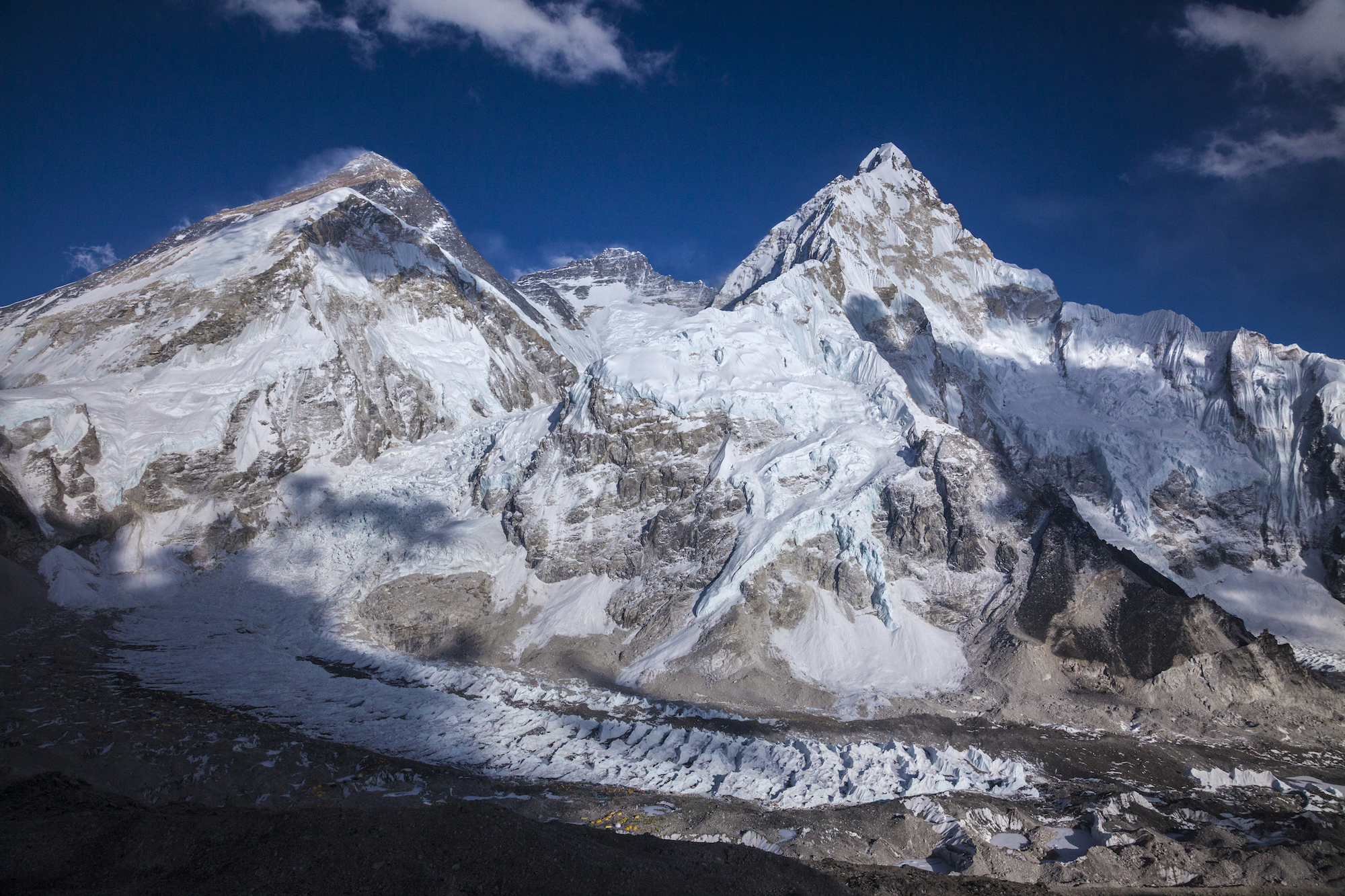A spectacular horizontal photograph captures an awe-inspiring mountainscape under a deep, rich blue sky, accented by a few wisps of clouds at the top. Dominating the frame are two prominent peaks just right of center, with a smaller peak nestled between them. A majestic glacier weaves through the narrow valley between the peaks, curving elegantly down the front of the left peak and wrapping around its base, extending towards the right mountain. The left side of the image is bathed in shadows, adding depth and contrast, while the foreground on the right reveals the rugged end of the glacier, juxtaposed against a stony, mountainous terrain. The intricate details and varied textures of the landscape draw the viewer into this breathtaking natural scene.